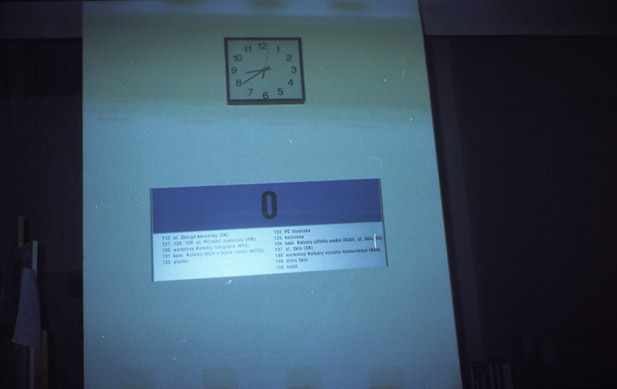The image features a white wall with a prominently displayed analog clock at the top center. The clock has a white face and a black border, showing the numbers 1 through 12. The second hand is pointing between the 1 and 12, the hour hand is positioned slightly past 8 towards 9, and the minute hand is on the 8. Below the clock, there is a large blue rectangle with a bold zero in the center. Surrounding this rectangle, there are numerous columns of text and numbers, likely representing data or information, with the most prominent column situated on the right side of the blue rectangle.